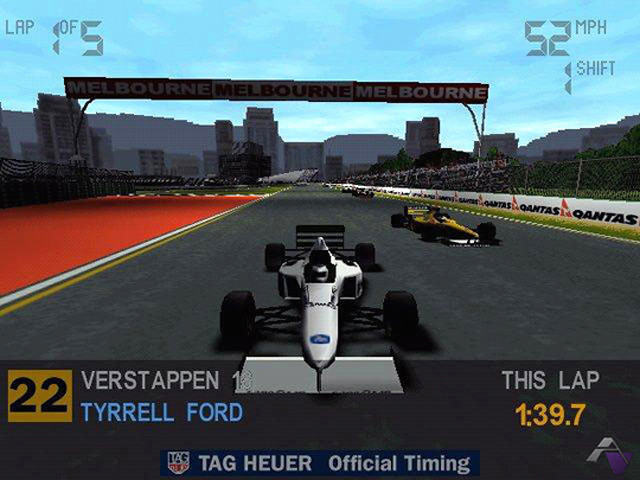This horizontal rectangular screenshot captures an intense racing game, seemingly set on a console or computer. The setting is a bright, daytime race track with a vivid blue sky. Dominating the center, a unique and sleek silver racing car is heading straight towards the viewer on a black road. This standout vehicle features four wheels spread apart from the main body of the car. Flanking the main car on the right are a yellow racing car heading towards the center and other smaller cars in the distant background. The background is bustling with a crowd in the bleachers, large city buildings, and hills with touches of greenery.

The track is adorned with various details, including a massive black rectangular banner hanging overhead, emblazoned with "MELBOURNE, MELBOURNE, MELBOURNE" in bold white capital letters. The left side of the track sports a bright red ground, while the right side is lined with a white wall marking "QANTAS" in bold black letters, accompanied by a red triangular logo repeated several times. Beneath the crowded bleachers are advertisements.

At the bottom of the image, a yellow block highlights the number "22" in black. Just above this block is the name "VERSTAPPEN" in gray lettering, and beneath it, "Tyrell Ford" in blue. Additionally, a royal blue rectangular bar at the very bottom contains the Tag Heuer logo followed by the words "TAG HEUER" and "OFFICIAL TIMING" in gray lettering. Towards the right side of the screen, there's an indicator showing "This Lap" in gray, followed by a timing of "1:39.7" in yellow. In the upper-right corner, the word "Shift" is visible, indicating a control command for the game.